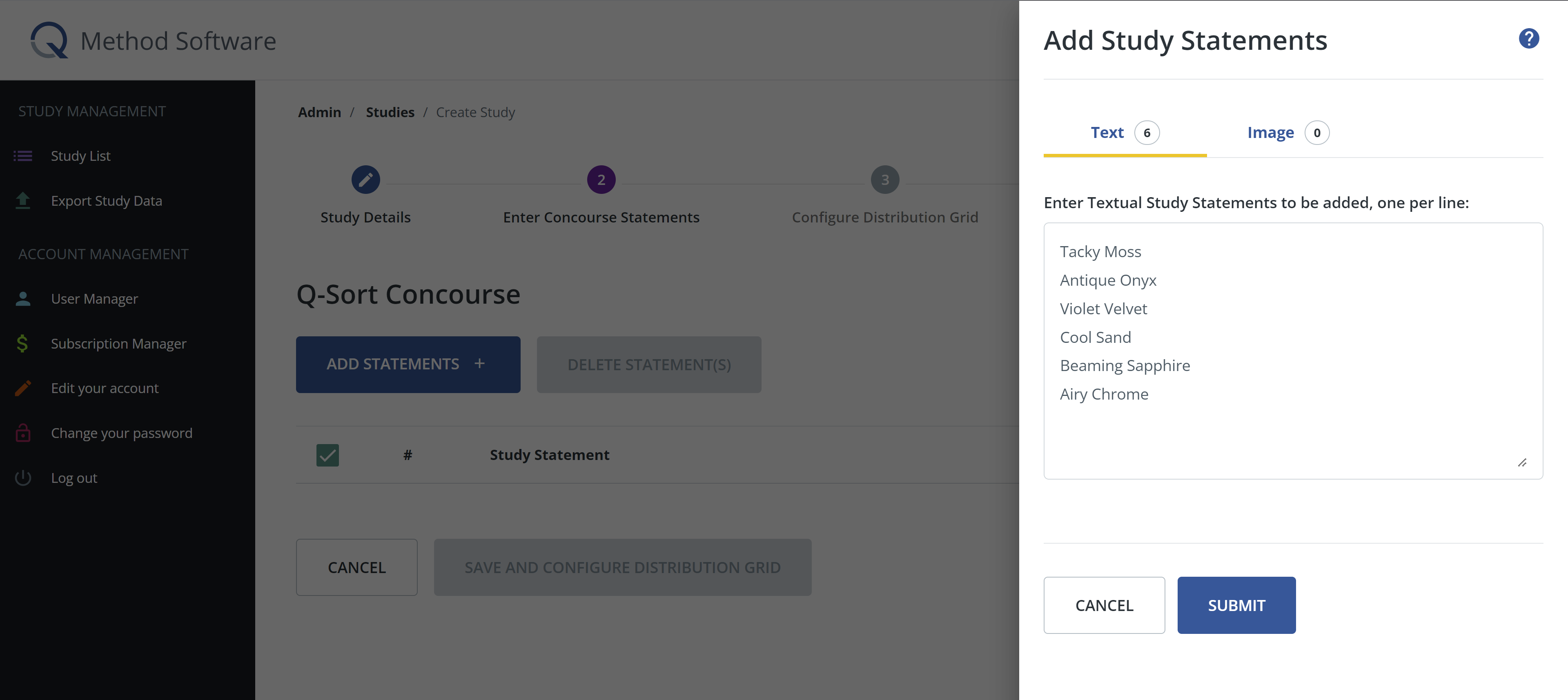The image showcases a detailed interface of a software named "Method Software." The interface is presented within a large, slightly grayed-out box, making some elements hard to read. At the top center, there is a circular icon with a line originating from its bottom right, forming a counterclockwise arc.

In the central part of the interface, a prominent black column block features the header "STUDY MANAGEMENT" in white, all-caps text. Below this header are several sections labeled as follows:
- "Study Lists" in white
- "Expert Study Guide or Data"
- "Account Management" with subsections like "Edit Your Account," "Change Your Password," and "Log Out"
- "User Manager"
- "Subscription Manager"

To the right of this main column, at the top, is a navigation path reading "Admin / Study / Create Study." Beneath this, there is a section titled "Study Details" marked with a pencil icon. This area contains a step-by-step guide:
1. Enter a Concourse of Statements
2. (Tasks not started) Configure Distribution Grid

Directly below the "Study Details" header on the left side, there's a subsection labeled "Q Sort Concourse." This area has functionalities:
- "Add Statements" indicated in blue with a plus symbol
- "Delete Statements" which is grayed out
- Options to mark statements with a checkmark for study or to cancel

Adjacent to this, an interactive section, brightly highlighted in white, displays a new box labeled "Add Study Statements" with a question mark icon. Underneath the label, a text field specifies the number "6" within a circled highlight. This area contains six underlined yellow sections titled "Image 0," prompting users to "Enter Textual Study Statements to be Added." Below this, there’s a list of sample options such as "Tacky Moss," "Antique Violet," "Velvet Pool," "Sand Beaming Sapphire," and "Any or Every Chrome." 

At the bottom of this interactive segment, there are two buttons:
- A "Cancel" button
- A "Submit" button in blue

This comprehensive interface is designed for efficient study management and detailed user account configuration.